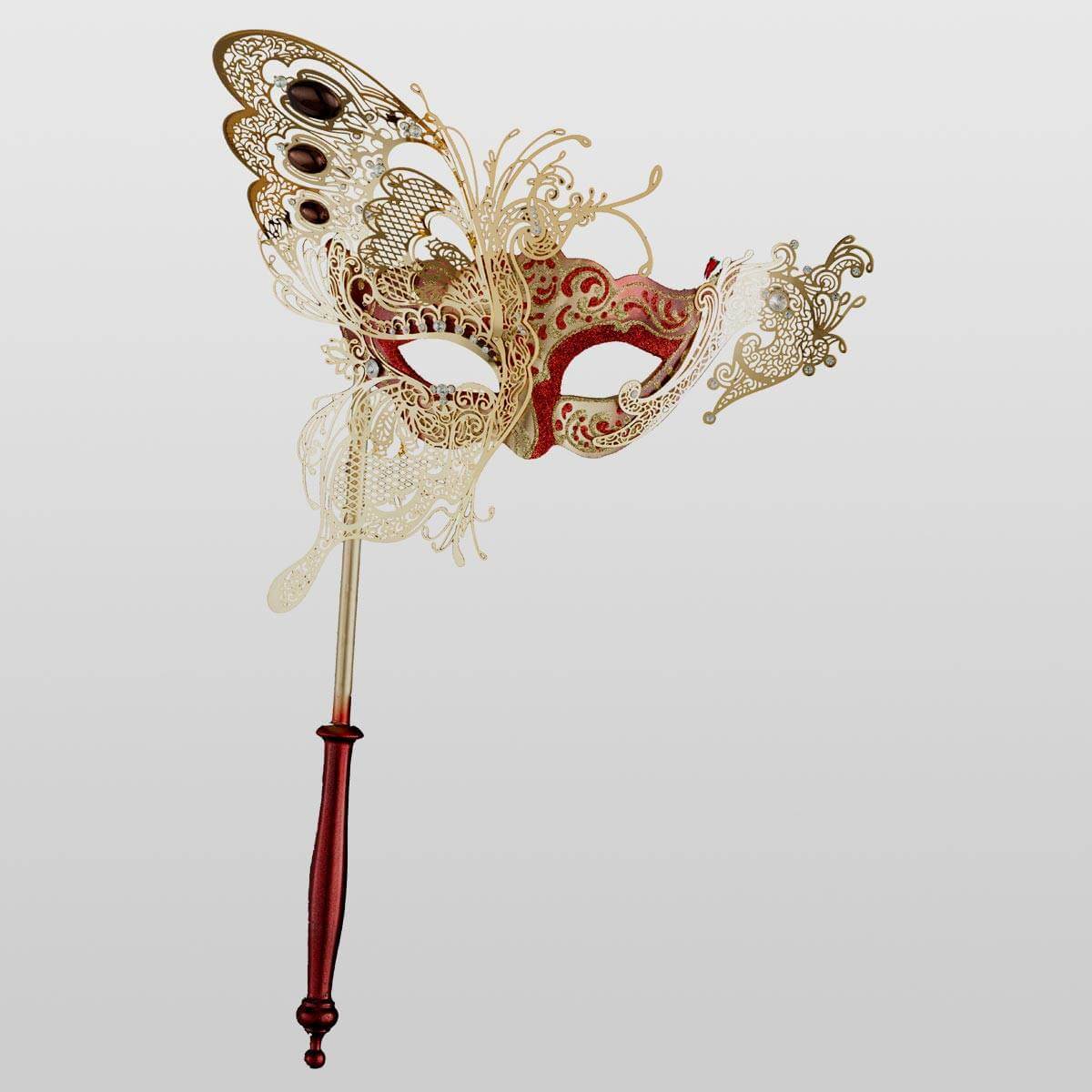The image depicts a professional photograph, possibly intended for use in a magazine or on a website for a costume store, showcasing a Venetian carnival mask. The mask, designed for handheld use, features a stick that transitions from cranberry red at the top to metal gold lower down, allowing someone to hold it comfortably in one hand. Set against a plain white background, the mask is poised elegantly, emphasizing its intricate and ornate design. Predominantly red and gold, the half-mask covers only the eyes and nose and is embellished with elaborate details, including delicate white lace at the bottom. On the left side, a striking feature that resembles butterfly wings with oval shapes extends outward, adorned in shades of brown, gold, and white, and further accentuated with black gems. The overall design is feminine and sophisticated, suitable for an elegant masquerade ball.